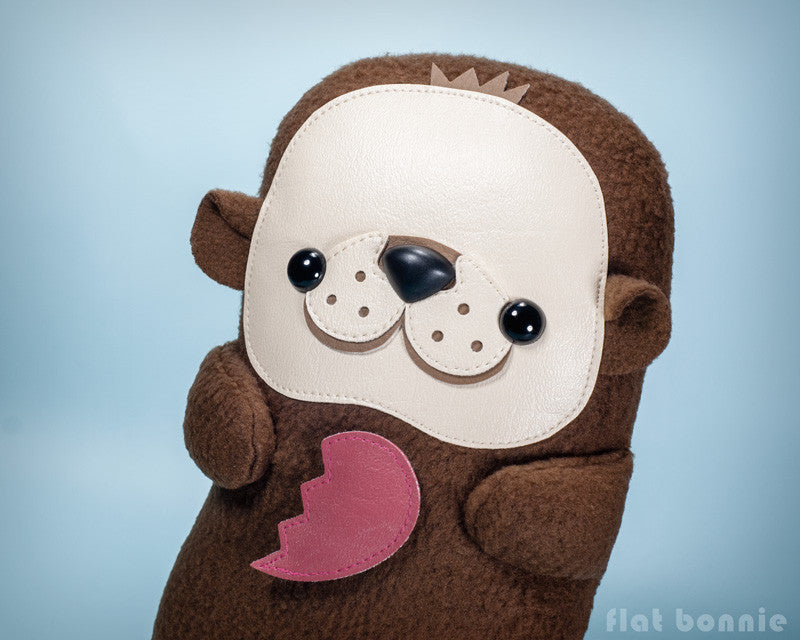This close-up photograph showcases an adorable stuffed animal resembling an otter or a bear, crafted from soft, brown plush fabric. The most striking feature is its face, made of cream-colored leather, creating a noticeable contrast against the felted body. The face is stitched on and features two large, hard plastic beads for eyes, and a black leather nose. The leather is cut to reveal some of the underlying beige-brown fabric around the nose and mouth area, adding to its detailed expression. The plushie also has small ears and tiny paws. On its chest, there is half of a red leather heart stitched on. The background is a light blue color, possibly indicating a wall. In the bottom right corner of the image, there's a watermark that reads "Flat Bonnie."